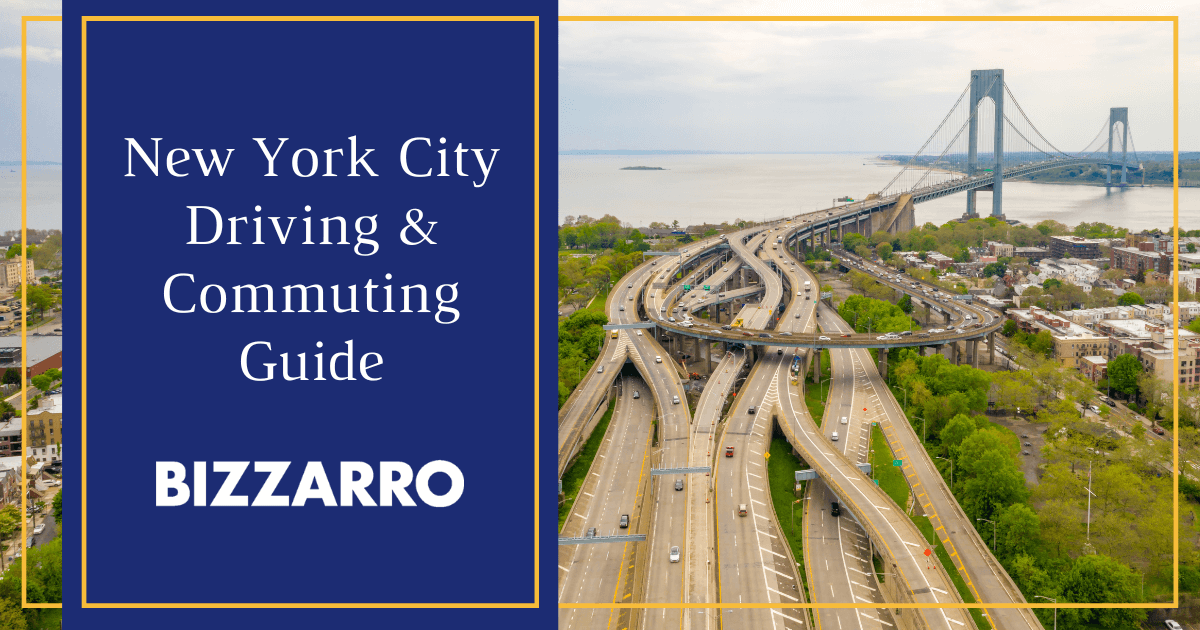The image resembles a book cover with a horizontally rectangular format. On the left, there is a vertically rectangular blue section bordered in gold, featuring white text that states "New York City Driving and Commuting Guide" and, in larger letters beneath, "Bizarro," which likely indicates the publisher. The right side of the image displays an aerial photograph of a complex network of highways in New York City, weaving together with some roads circling around and converging towards a prominent suspension bridge that spans a body of water such as a river or harbor. The scene is enhanced with digital effects and shows a cloudy sky and commercial brown brick buildings on the right. There are trees and greenery scattered among the roadways, and the highways include various diamond-shaped turns and multi-level lanes, adding to the overall complex and daunting appearance of the traffic system. The background further reveals more buildings and water, contributing to the intricate cityscape.